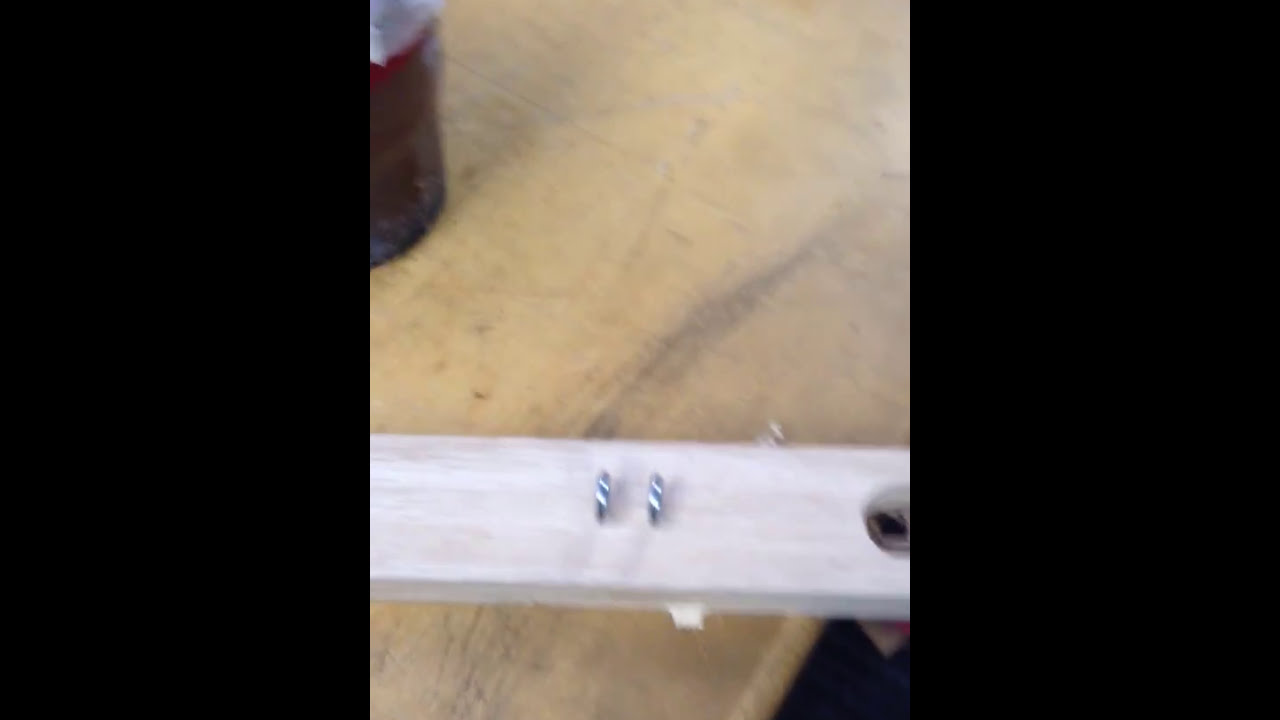The image depicts a blurry scene centered on a light gray wooden plank placed horizontally on a dark brown, scratched and well-worn workbench. The wooden plank has two thin metal rods inserted vertically and a semi-circular hole drilled on the right side. The blurred background includes an indistinct object in the upper left corner that appears brown with a possibly white top. Additionally, a red item, which could be a bottle or machine, is noticeable, suggesting this may be a work or school setting. The predominant colors in the image are the yellowish-brown of the table, the white and silver of the plank and metal components, and the red in the background.